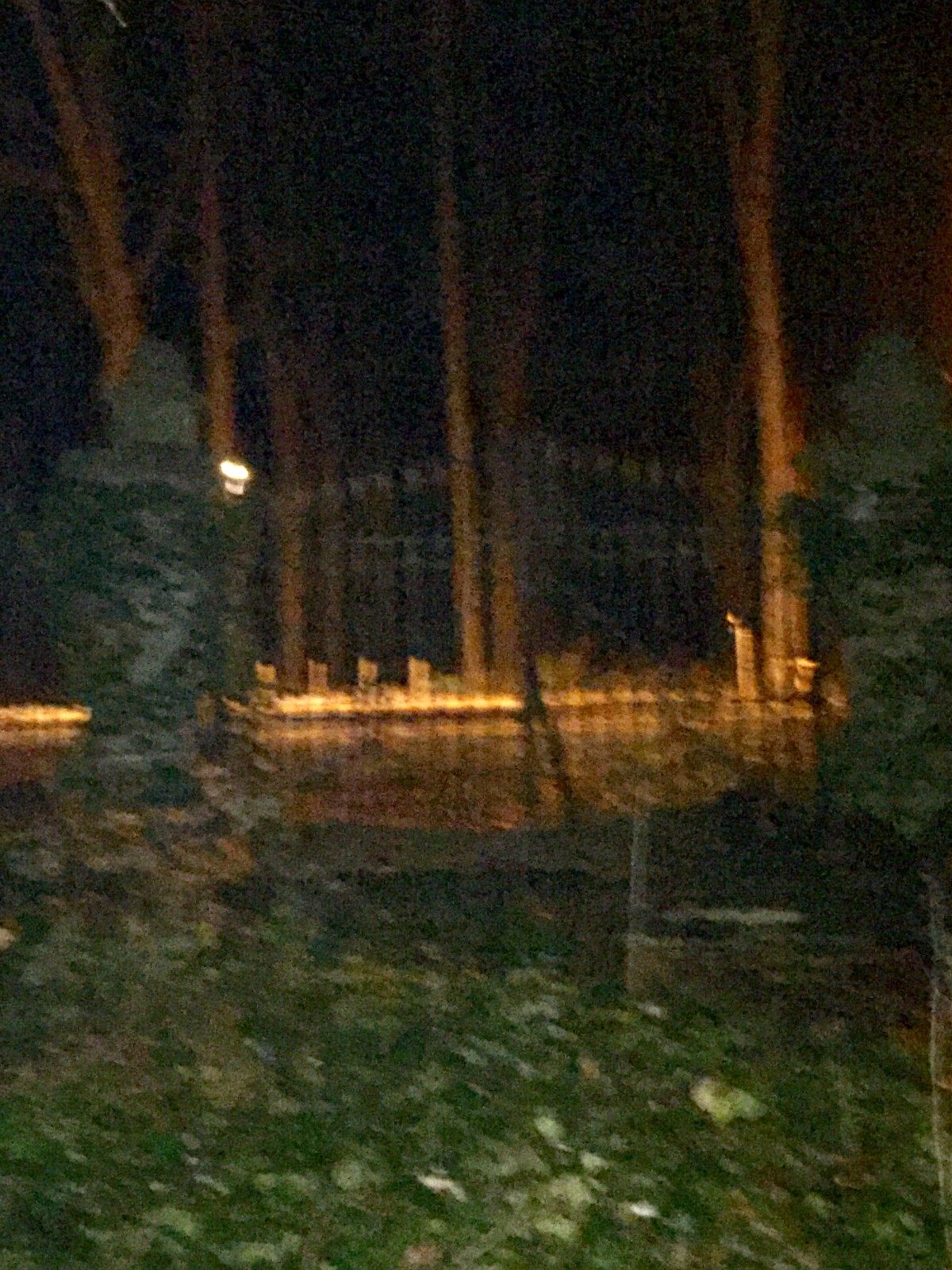The photograph captures a serene nighttime scene in nature, centered around a small, closed fence. The fence, which appears to be black or a dark color, contrasts subtly against the dim background. Flanking either side of the fence are two tall fixtures adorned with greenery, adding a touch of life and texture to the composition. The ground beneath the scene is covered with grass, with a few flower petals scattered about, suggesting a lush, natural setting. In the distance, a streetlight casts a gentle glow, providing the only artificial illumination in the otherwise dark night. The entire area is surrounded by tall trees, reinforcing the feeling of being enveloped by nature. The open, expansive space, combined with the darkness of the night, gives the image a tranquil yet mysterious atmosphere.